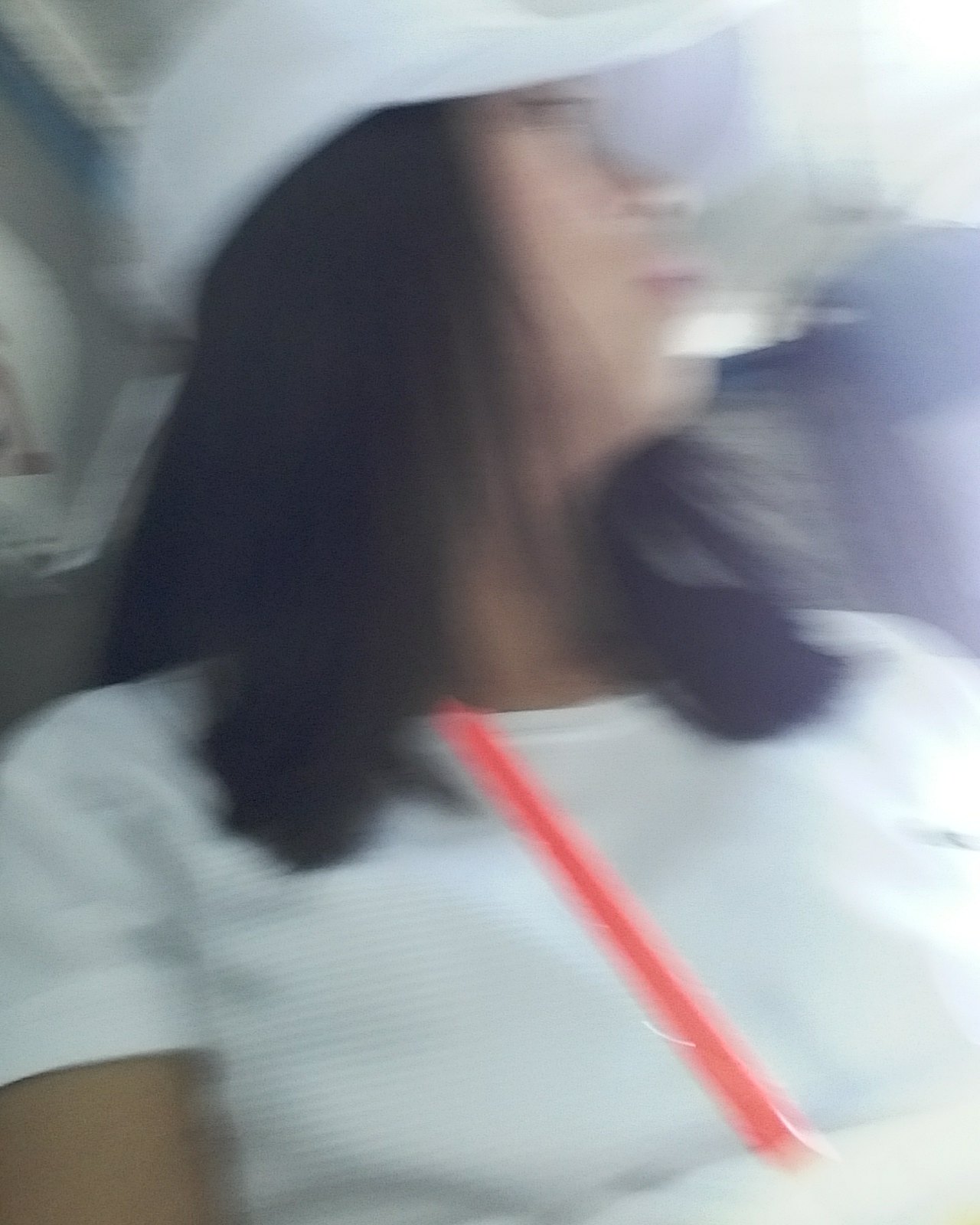In this slightly blurred photograph, a woman with shoulder-length black hair is captured. She is wearing a white baseball cap adorned with a green logo on the top right corner near the equivalent of a breast pocket area of her white t-shirt. A red strap, presumably from a crossbody bag, runs diagonally across her chest. The backdrop of the image suggests she is seated, either on a blue chair or perhaps on public transit with blue seating. The photograph, taken from a low angle near her midsection and facing upwards, provides an under-the-chin perspective as she tilts her head to her left, gazing into the distance and avoiding direct eye contact with the camera.